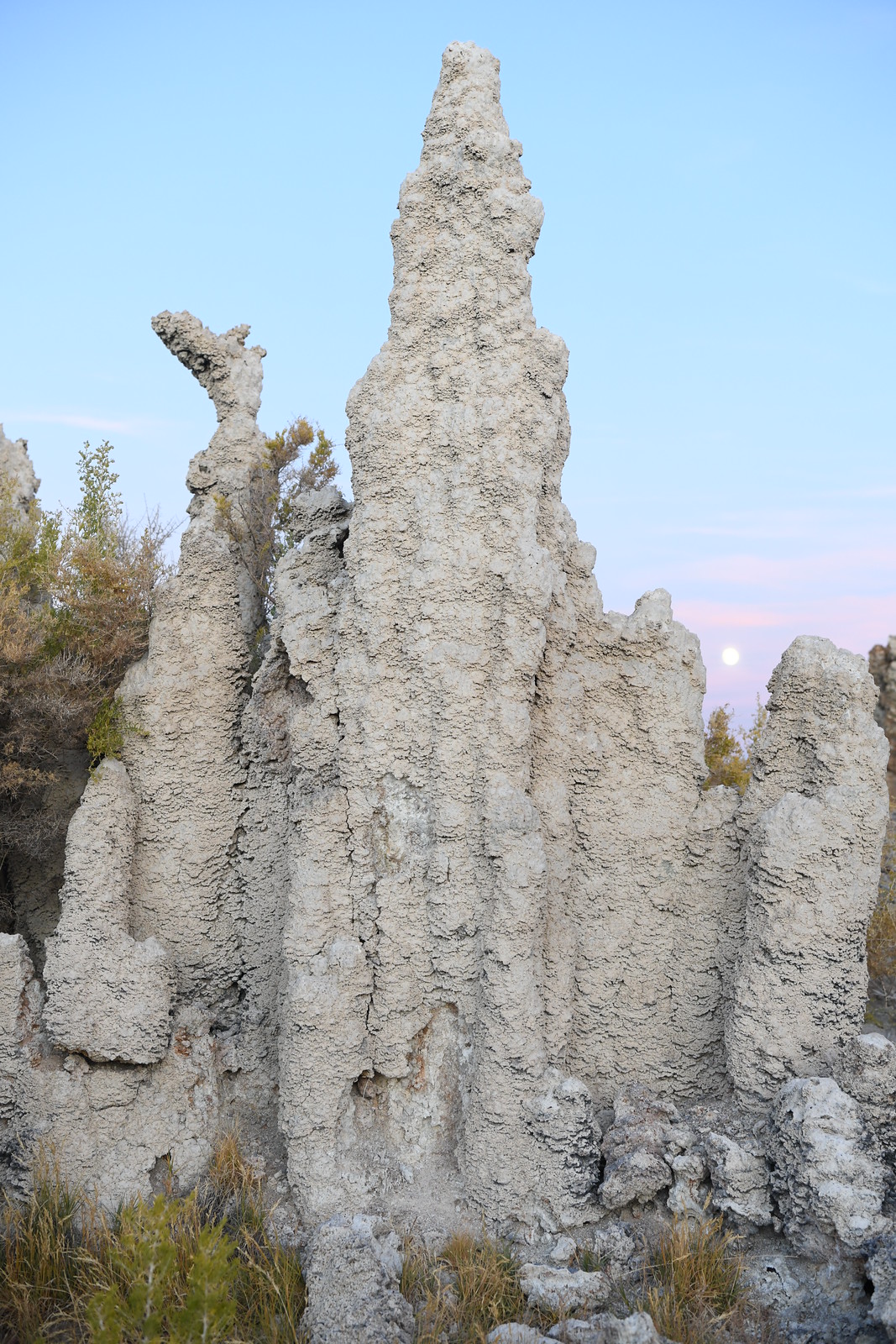The photograph captures a striking and detailed scene of a tall, uniquely structured rock formation, reminiscent of a termite or ant mound. The rock formation consists of several pale white and light gray pillars that range up to an impressive 28 feet, the tallest peak standing prominently among the smaller ones. Surrounding the base of this formation is a sparse covering of dry, light green and brown grass, mingling with golden weeds and plants, suggesting a desert-like environment. In the background, similarly hued trees and bushes enhance the rugged, natural setting. The sky above is a vivid light blue, with hints of pink from the setting sun, which is visible as a soft, round white circle on the horizon. The entire image exudes clarity and brightness, typical of a well-lit outdoor scene, devoid of any human-made elements, immersing the viewer in its serene and untouched beauty.